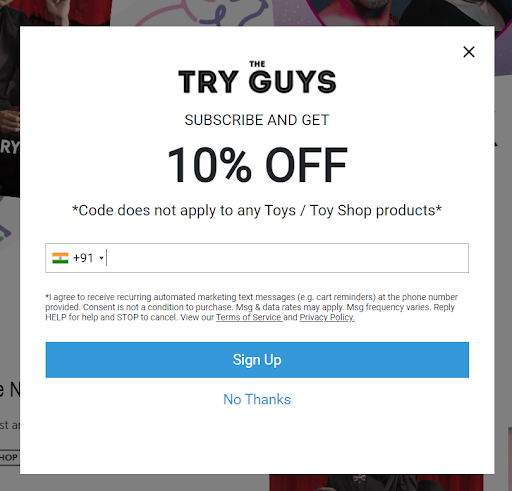The image appears to be a screenshot of a web page. The background is obscured by a large white overlay with a very thin border. On this white overlay, in bold black text, are the words "The Try Guys Subscribe and get 10% off." Beneath this, there’s a smaller note that reads, "Code does not apply to any toy shop products."

Below the text, there is a long input bar featuring an icon of a flag with three horizontal stripes in orange, white, and green, which is the flag of India. Next to the flag icon, it says "+91" followed by a divider and then an empty space designated for entering a phone number.

Below this input bar, a disclaimer states: "I agree to receive recurring automated marketing text messages including cart reminders at the phone number provided. Consent is not a condition to purchase. Message and data rates may apply. Message frequency varies. Reply HELP for help and STOP to cancel. View our Terms of Service and Privacy Policy."

At the bottom of the overlay, there is a long blue button with the text "Sign Up." Below this button, there is a clickable option that says "No, thanks."